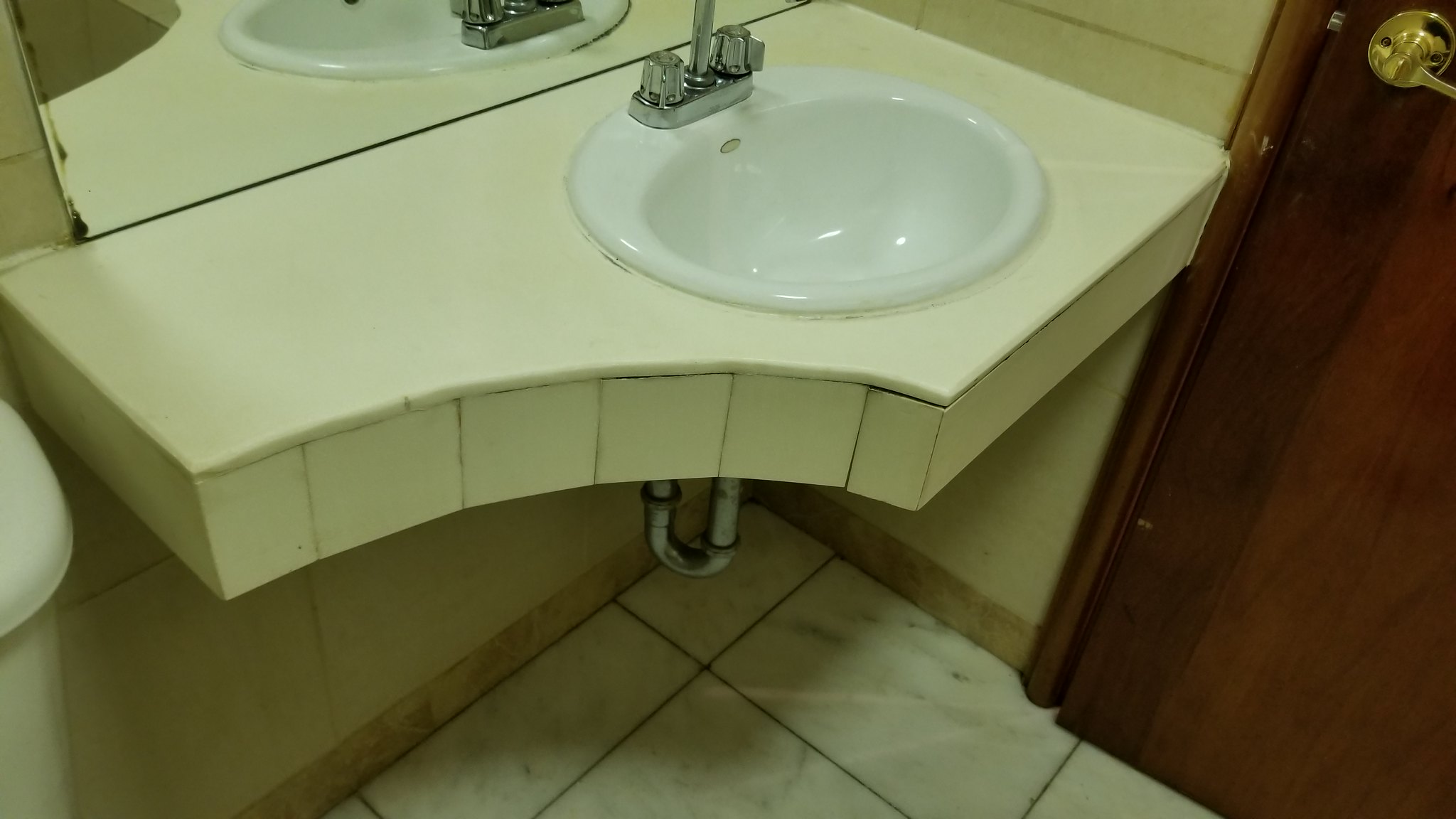The image captures a vintage-style bathroom with a distinctly old and slightly dingy ambiance, reminiscent of a scene from a thriller movie due to its yellowy-green hue. Central to the photo is a prominent white porcelain sink with silver fixtures, projecting from the wall. The sink, mostly rectangular with a unique curved corner, is complemented by a small counter that mirrors its arc, decreasing counter space while boosting floor space. The countertop is somewhat plain beige with noticeable tiling along its edge.

Beneath the sink is a visible silver pipe connecting to the wall, reinforcing the aged and utilitarian aesthetic. The surrounding walls are lined with tan-colored tiles, their grout notably dark and worn, lending an air of neglect despite the cleaner appearance of the tiles themselves. The floor contrasts with its white or light gray granite-like tiles arranged in large squares.

To the right, a dark wood-grain door with a golden handle hints at the room's overall warmth in color tone. Partially visible at the photo's left edge is the top of a white porcelain toilet, cropped out of full view. A mirror behind the sink adds depth to the image, reflecting the space and enhancing its vintage charm. Overall, this small, timeworn bathroom emanates an old-fashioned and slightly eerie atmosphere.